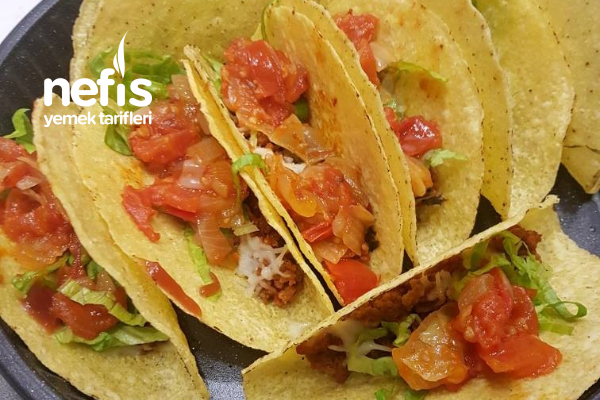This color photograph beautifully captures a tantalizing arrangement of tacos, presented from an overhead view. The tacos, enclosed in crispy, light brown shells with subtle brown specks, are meticulously arranged on a dark black plate with a sophisticated ribbed pattern on its edge, interspersed with white speckles. There are six tacos placed across the plate, forming a central row, flanked by one additional taco on each end of the row, making a total of eight tacos. The shells are generously filled with vibrant ingredients, including red chopped tomatoes, possibly some onions or chives, green leafy lettuce, savory meat, and a sprinkling of white cheese. The plate is set against a stark white surface, creating a striking contrast that highlights the vivid colors of the taco fillings and the yellow hues of the taco shells. The text "Nefes Yemek Tarifleri," suggesting a different language, adds an international touch to the composition, which could be situated in either a kitchen or a restaurant setting.